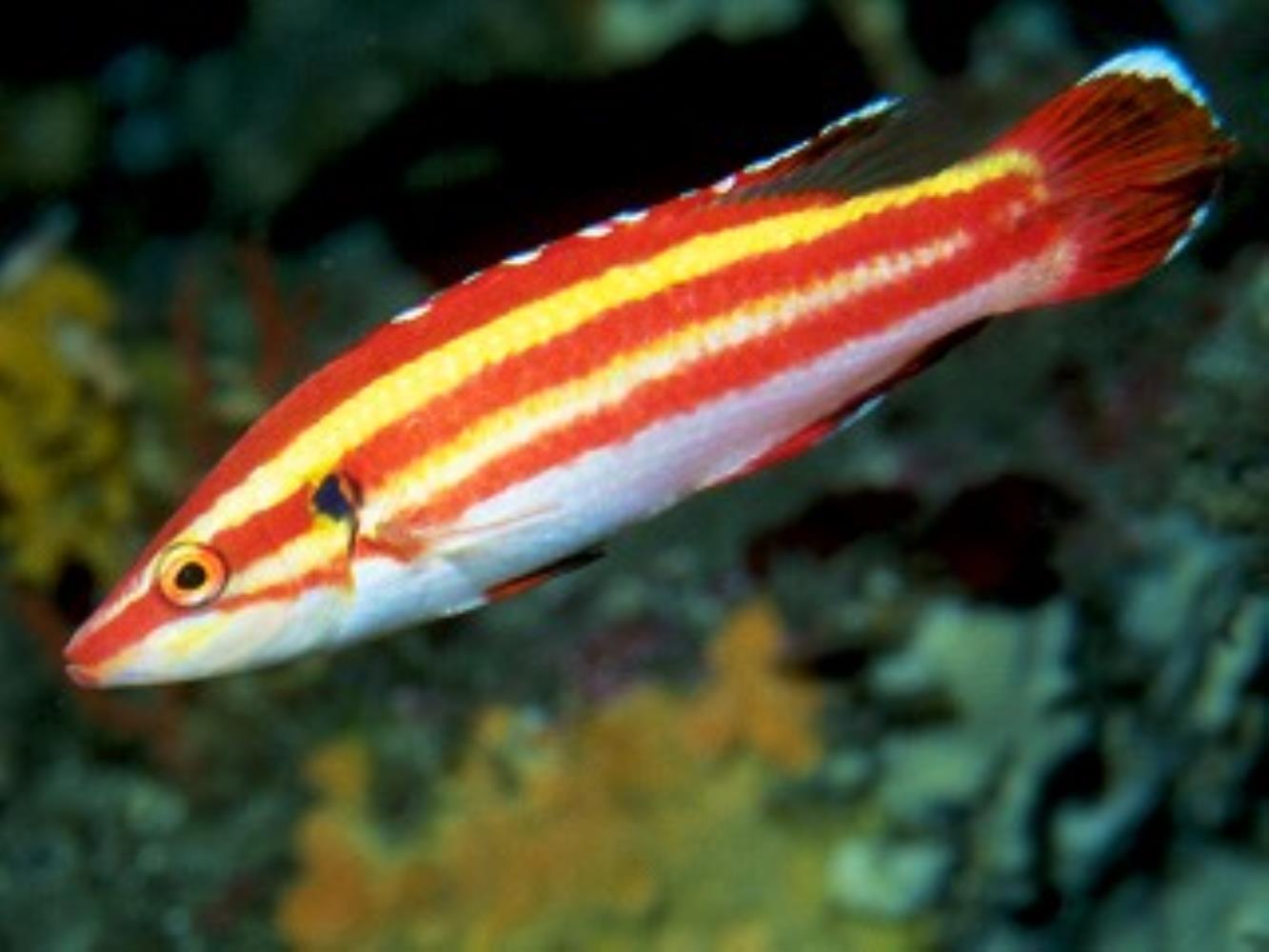This detailed close-up photograph captures a small fish vividly swimming in water, with its mouth aimed toward the bottom left and its tail extending to the upper right corner of the image. The fish is adorned with striking red, orange, and white stripes running horizontally across its body, with some stripes evolving into a yellow hue. Its round eyes, primarily black with a subtle yellowish-orange tint, give it a distinctive appearance. The fish also boasts red fins and a red tail, both of which are accented with white tips. The blurred background, likely the bottom of the sea or a lush aquarium, features various colors and shapes, including hints of yellow and blue, indicating the presence of aquatic plants or other underwater structures.